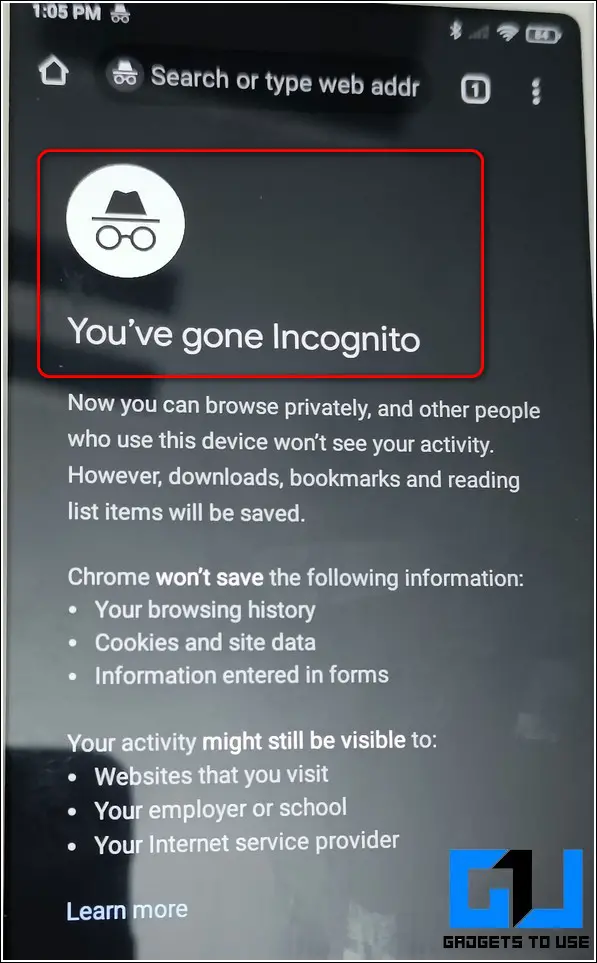This photo captures a grainy, real-life image of a mobile device's screen, showcasing a series of activities and edits. The entire frame is dominated by the phone screen, with only a small portion of the neutral white background visible in the top right corner. 

At the top left of the screen, the time is displayed as 1:05 PM in white text. To the right of the time, the incognito mode symbol is visible. Further along the status bar, there is an empty space before the Bluetooth symbol, an indicator showing zero cell signal bars with a small 'X', a white Wi-Fi icon, and finally, a battery indicator showing 84% charge.

The display below reveals the browser, which is Google Chrome in dark mode. The upper section of the browser shows a home icon on the far left. Next to it is the incognito symbol within the URL bar, indicating an incognito session. The URL bar contains the truncated text "searcher type web ADDR" and ends with a rounded square featuring a '1' and a three-dot menu icon.

The main content area of the browser displays the incognito splash screen. There’s a central incognito symbol in black within a white circle, with the text "You've gone incognito" below it. This area is highlighted by a red rounded rectangle, an edit made by the user. Additional text providing information about incognito mode lies below this highlighted section.

In the bottom right corner, the user has added a watermark featuring a combined blue and black "G" and "U" logo, labeled "gadgets to use."

Reflective details reveal part of the surrounding environment where the photo was taken. The bottom left corner shows the edge of another device used to capture this image, while the reflection discloses portions of the ceiling or wall, which are white, and unidentified black shapes that might be elements like a ceiling fan, furniture, or window.

Overall, the image is a multi-layered snapshot of a mobile phone screen in incognito mode, annotated with edits and contextual room reflections.